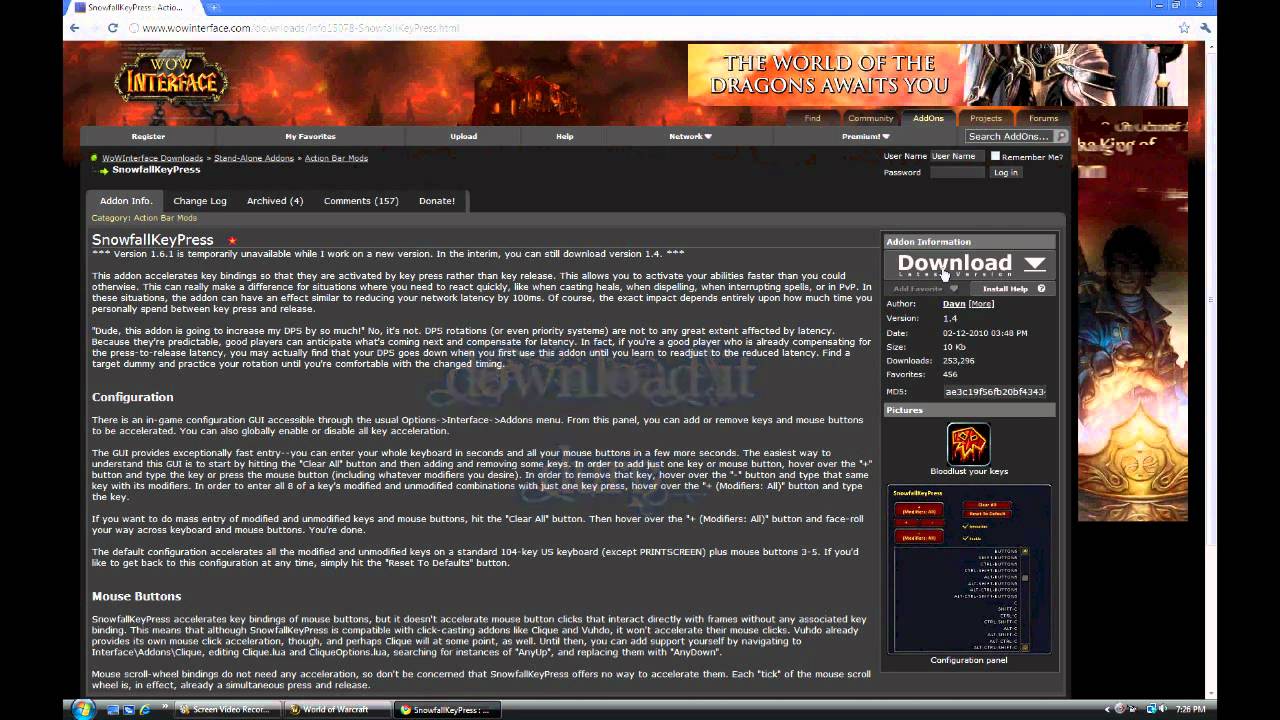The screen capture appears to be from a gaming-related website, but the text is extremely blurry and mostly illegible. At the top, a white address bar is visible with a black web address. Common browser icons such as the back, refresh, star, and wrench icons are identifiable. Additionally, there's a thin blue strip with a minus sign and the tab name.

In the background, a fiery battle scene dominates the upper section. This includes vivid orange and black colors highlighting a building engulfed in flames. A medieval-themed logo reading "Wow Interface" is noticeable, with its wooden design and orange font. A prominent banner declares, "The world of the dragon awaits you," set against an orange, fiery backdrop. Adjacent to the banner, there's an image featuring brown and gold armor.

Moving down, menu tabs with difficult-to-read text in a brown and gold color scheme can be seen, suggesting options like "feed" and "add-ons." A search box is also present. Further down, an ad displays a magician-like figure in a blue coat, reaching out towards the viewer with a golden orb near his hand. Below this ad, a gray box with "download" in white text is visible, featuring an orange and red image.

Continuing down the page, a lengthy blog post titled "Snowfall Key Press" is present, containing several paragraphs of text. Finally, gray tabs with white font are visible, and at the bottom of the screen, a Windows icon, more open tabs, and a clock can be seen.